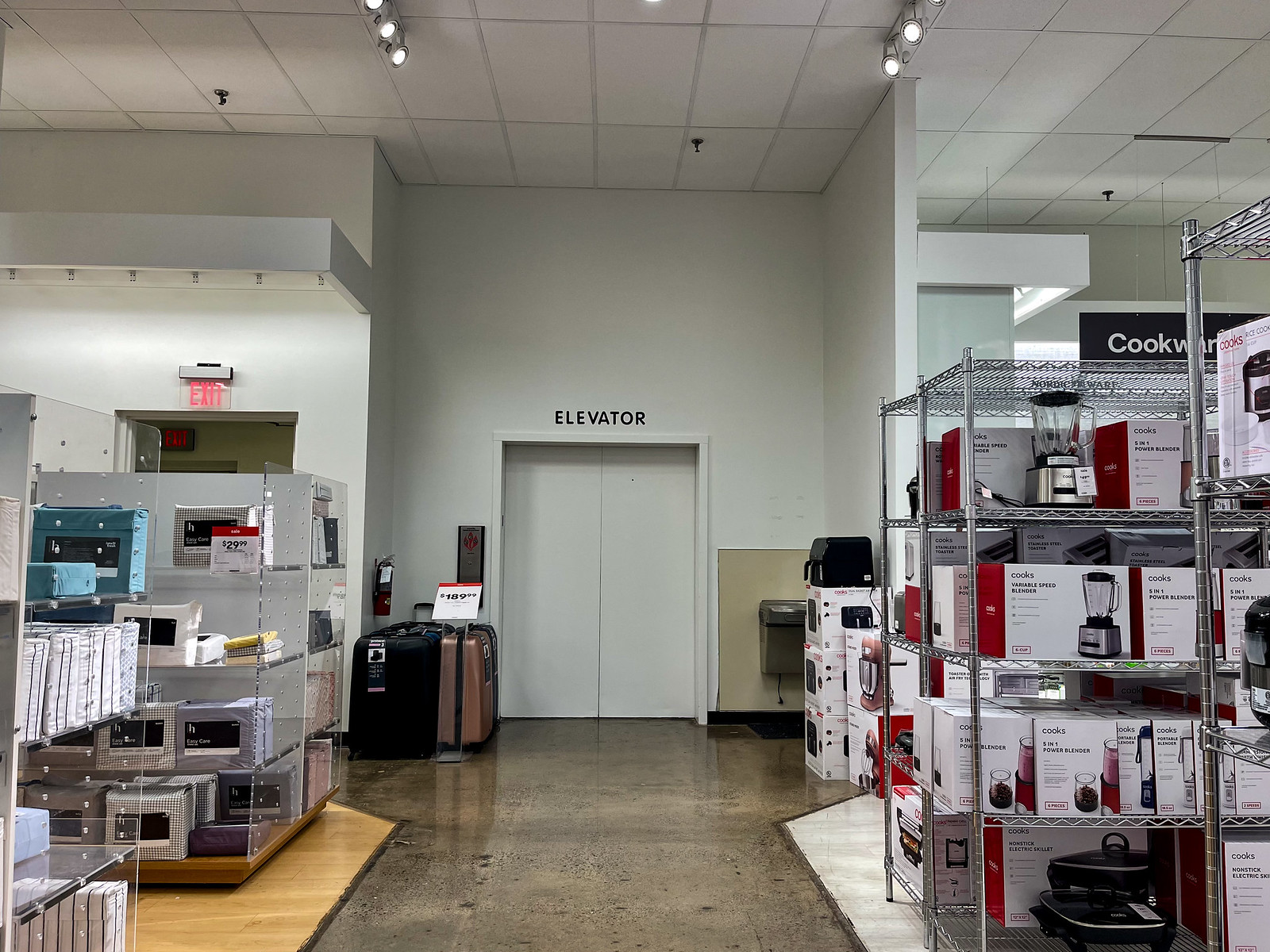The photograph captures the interior of a meticulously organized and well-stocked appliance store. In the center of the image, a clearly labeled white elevator stands against a beige wall, with a water fountain to its right and a fire extinguisher to its left. Next to the elevator, display shelves hold an array of luggage priced at $189.99. To the right, under a sign labeled "Cookware," shelves are filled with a variety of blenders. To the left, shelves display microwave ovens and packages of bedding neatly arranged in cube forms. The floor of the store is made of shiny brown marble or tile, adding to the polished look of the environment. An exit sign is visible in the back left, guiding customers to the store's exit.